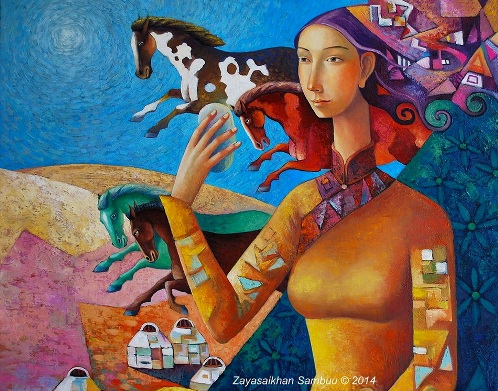This semi-abstract, surrealist painting, copyrighted in 2014 under the font inscription "Zaya Saikan Sanbul," depicts an elongated white woman set against a dreamlike outdoor landscape. The woman, who wears a high-collared brown dress accented with triangular patterns, has a strikingly elongated neck, nose, and fingers. Her black hair is partially concealed by a rich purple and red headscarf. She holds an oval, possibly phone-like object in her extended hand, bent back towards her face.

Surrounding the woman are several vibrantly colored, surreal horses. To her left, there are blue and black horses, while above and to her right are a spotted brown-and-white horse and a darker brown horse. Another set of horses appear in various hues including red, green, and blue, some adorned with white dots, seemingly moving or flying across the landscape.

The background features a blue sky with rolling hills shaded in pink, purple, and brown, creating an abstract, undulating terrain. Dotting the ground below are whimsical, small structures resembling milk cartons with little domes. The scene includes a variety of geometric patterns and shapes, adding texture and layers to the vividly imaginative composition.